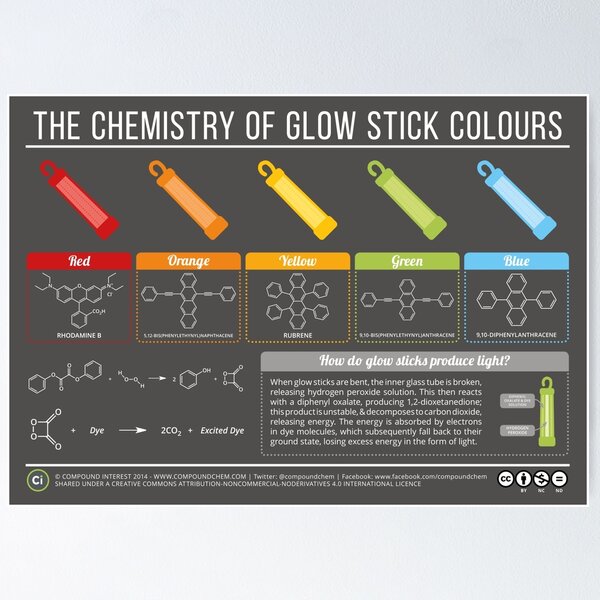The image is an infographic against a brown background, emblazoned with the title in white font: "The Chemistry of Glowstick Colors." Beneath the title are five glowsticks, each showcasing a different hue—red, orange, yellow, green, and blue. Directly below each glowstick, chemical designations specific to the color are displayed. A key section in the lower right corner explains the science behind glowsticks: bending a glowstick breaks its inner glass tube, releasing hydrogen peroxide, which reacts with diphenyl oxalate to produce 1,2-dioxetanediode. This unstable compound then decomposes to carbon dioxide, releasing energy absorbed by dye molecules. Electrons in the dye return to their ground state, emit excess energy as visible light. The image footer includes licensing information from Compound Interest, 2014, with its logo, Twitter handle, and a Creative Commons license detail.